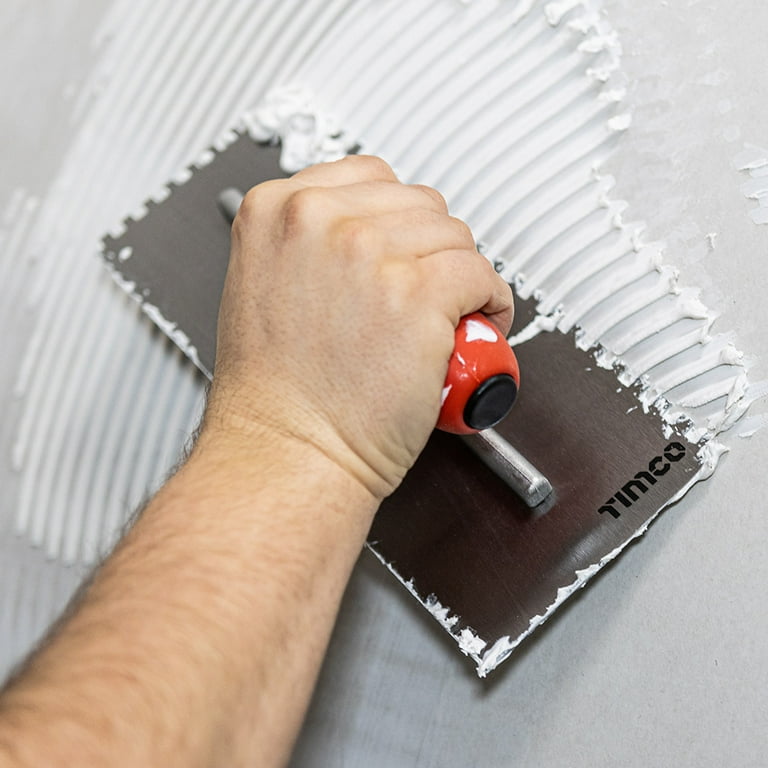In the photograph, a white man is seen using a flat metal tool with a serrated edge and a red plastic grip to spread a substance—likely grout, plaster, cement, or paint—onto a light gray wall. The tool, which bears the logo "Temco" in the lower right-hand corner, is held firmly as it creates a striped pattern on the surface. The man appears to be engaging in construction or tiling work, carefully evening out the material to ensure a smooth application. The background suggests a typical construction setting, with a light gray, cement-like surface that could also be sheetrock.